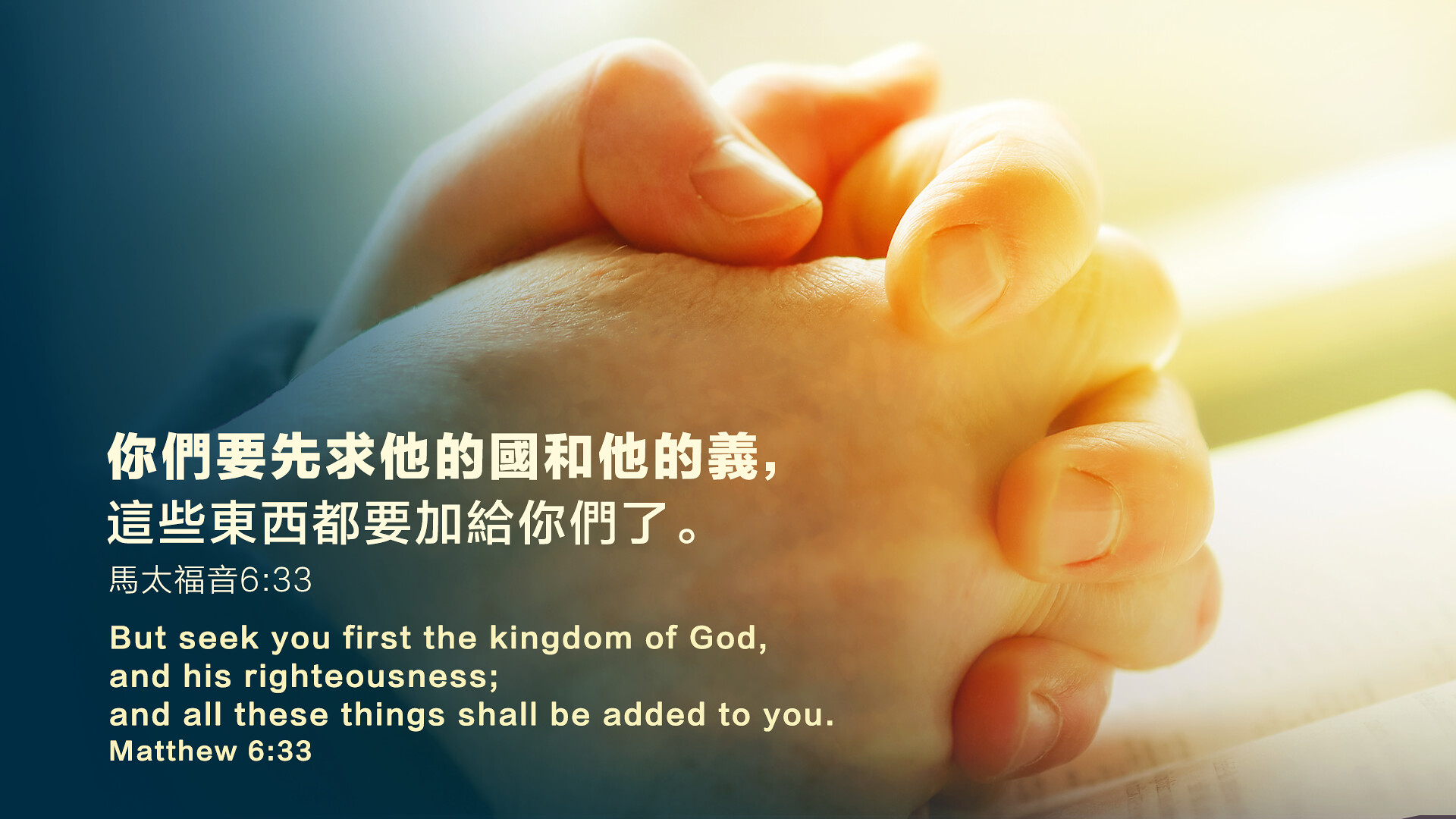The image depicts hands resting on an open book with fingers interlocked in a gesture reminiscent of fervent prayer. The book, likely a Bible, sits beneath the hands, visibly open to a specific page. Above the hands, the image displays three lines of Chinese characters, while below them, an English translation reads, "But seek ye first the kingdom of God, and his righteousness, and all these things shall be added to you. - Matthew 6:33." The photo features a contrasting color gradient, transitioning from a dark blue on the left side to a bright yellowish-white on the right, emphasizing the light source that appears to illuminate the scene. This thoughtfully constructed image serves as an inspirational meme, combining religious text in both Chinese and English to reinforce a powerful biblical message.